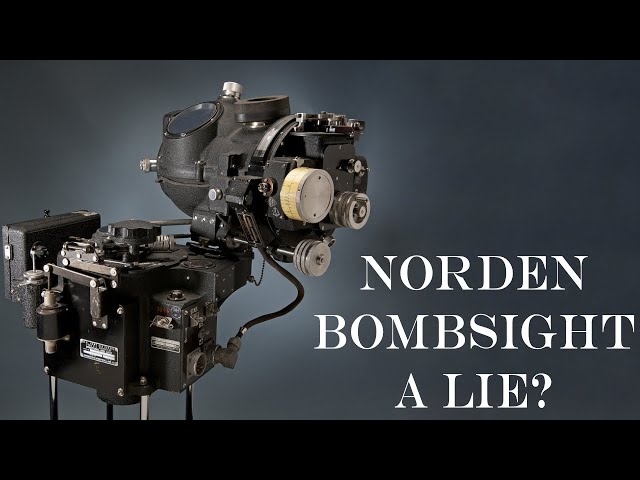The image depicts a complex and detailed piece of machinery, predominantly black with sections of chrome. The equipment stands tall on four supports and features a series of interconnected parts and lenses, some with caps on them. In the background, there's a large black box and the overall setting is framed by a black border with a gray backdrop, though some descriptions mention a cloudy blue background. The machinery has various metal components, possibly cast iron, along with numerous pipes, tubes, and screws, hinting that it might be related to aviation. A label on the equipment reads “Norden bombsite a lie?”, suggesting it might be a bomb sight. The image blends a computer-generated elements with a photograph and includes white text on the right side.